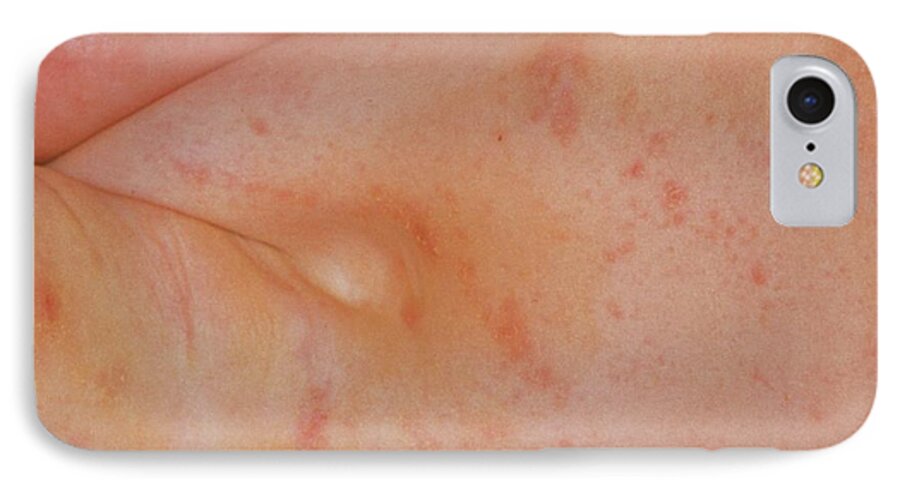The close-up image, likely taken with a mobile phone, depicts white skin covered in red splotches and small sores indicative of a mild rash. The exact body part shown remains ambiguous due to the proximity of the shot. Notably, a white plastic element, possibly resembling a mobile phone camera and flash, is visible in the upper right corner, which could suggest the image was either captured on or edited with a phone. This white plastic detail stands out against the peach-colored skin, contributing to the image's peculiar composition. The photograph seems intended to document the skin condition for medical consultation, such as with a dermatologist, given the clear and focused depiction of the rash.